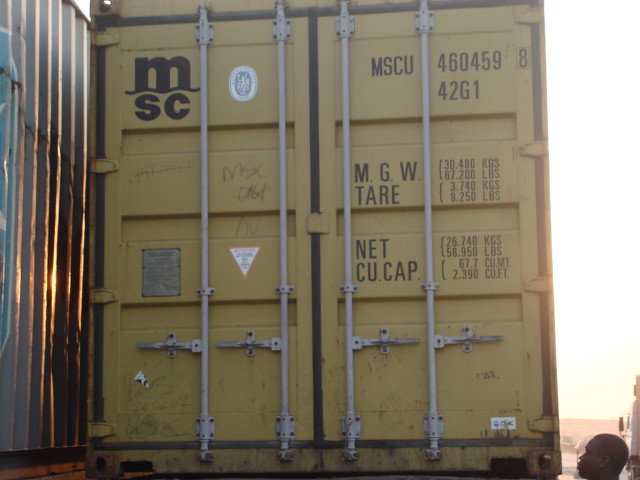The image features the back of a yellow shipping container commonly seen on large freighters near the ocean. The prominent yellow container, which is surrounded by a tiny portion of a white container on the left side, dominates the scene. This yellow container is marked with the logo MSC: the letter "M" styled with an ocean wave design, followed by the letters "SC" underneath. The numbers "460459" and "42G1" are also visible, along with "MGW 30,480 kg" and "net CU cap 26,740 kg." Additionally, there's a warning sticker shaped like an upside-down triangle. Four containers are stacked, but only the bottom two and the lower part of the top two are visible in the photo.